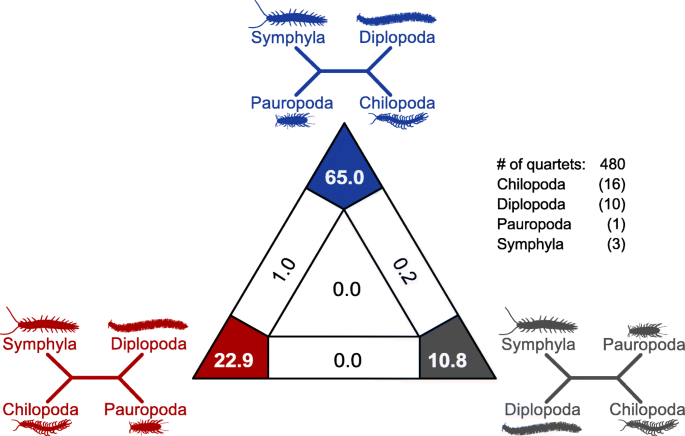The image is a detailed scientific diagram featuring various arthropods. At the center of the diagram is a large triangle segmented with lines, and within this larger triangle is a smaller, inset triangle. Positioned at the vertex of the upper tip of the large triangle is a blue diamond shape, labeled with the number 65.0. The bottom left tip of the triangle is red, marked with the number 22.9, while the bottom right tip is gray, showing the number 10.8. Along the edges of the triangle, numbers such as 1.0, 0.2, and 0.00 are displayed respectively.

Above the triangle, there are shadow drawings of four arthropods: Symphyla, Diplopoda, Paropoda, and Chilopoda, appearing to be connected in a manner akin to a chemical structure. These names and insect shapes are color-coded and repeated in blue, red, and gray text around the diagram: blue text at the top, red at the bottom left, and gray at the bottom right.

On the bottom right, additional text notes essential numerical data: "Hash of quartets: 480," and the names of the creatures with corresponding numbers in brackets—Chilopoda (16), Diplopoda (10), Paropoda (1), and Symphyla (3). This instructional image, designed to indicate interrelationships and classifications among the insects, uses distinct color coding and segmented parts with specified numbers to present detailed scientific information.